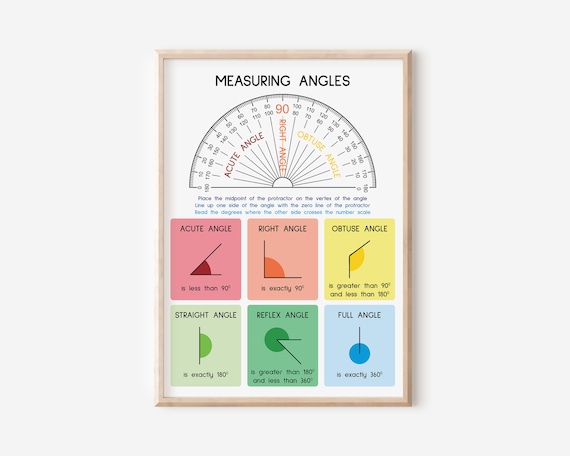A framed picture, set on a light brown wall, features a light brown wooden frame. At the top of the illustration, against a white background, there's black text reading "Measuring Angles." Below this text is a semi-circular protractor scale, resembling a half-circle compass, marked with degrees from left to right. On the left side of the protractor, the term "Acute Angle" is inscribed in orange, while the right side reads "Obtuse Angle" in yellow, and directly at the top center, "Right Angle" is labeled with "90" above it.

Underneath this scale, there are six squares organized in a 2x3 grid, each with different background colors and corresponding angle descriptions. The top row includes a pink square labeled "Acute Angle" with an illustration of an acute angle, an orange square labeled "Right Angle" with a right angle illustration, and a yellow square labeled "Obtuse Angle" with its respective illustration. The bottom row comprises a green square labeled "Straight Angle," a dark green square labeled "Reflex Angle," and a blue square labeled "Full Angle," each presenting a visual example of the respective angles.